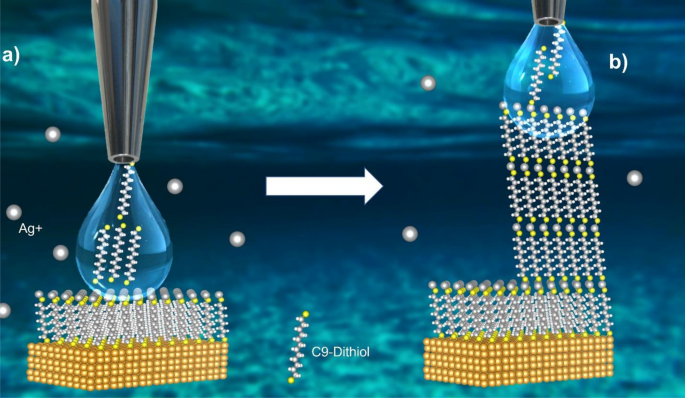The image is a detailed scientific illustration that resembles diagrams found in chemistry or science textbooks. The background features a gradient of blue to dark blue, giving it an underwater appearance. On the left side, labeled with a lowercase "a," there is a pipette or eyedropper releasing a droplet of water onto a cluster of cubes and small white spirals that resemble DNA or slinkies. In the center, a white arrow points to the right, indicating progression. On the right side, labeled with a lowercase "b," the white spiral structures are now neatly stacked four high and six across, with the water droplet positioned just above them. Chemical notations including "Ag+" (silver) and "C9" are included, adding to the diagram's scientific context and complexity.